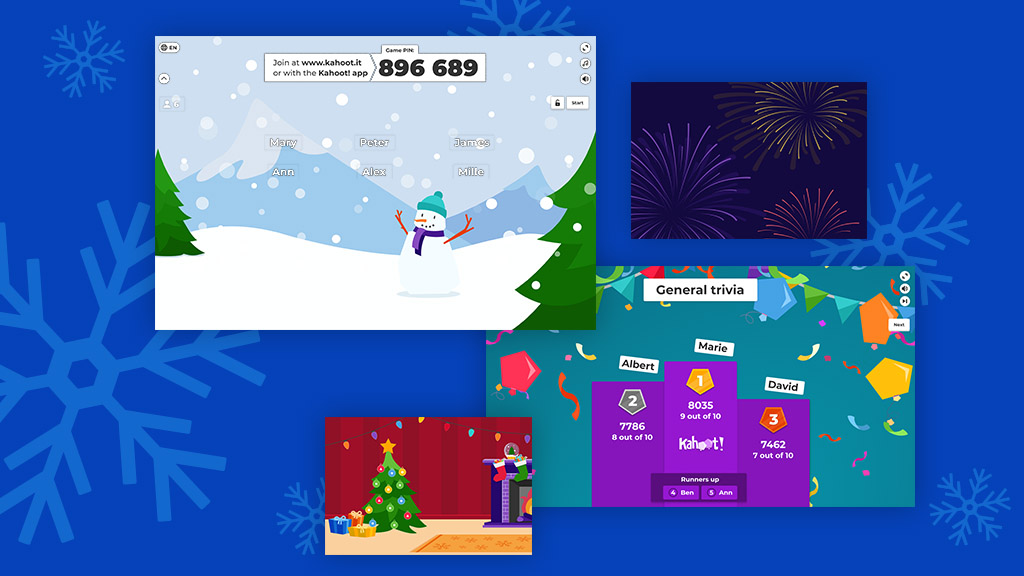This image is of a trivia page that appears to be a cutout. The top left section features an image of a snowman, and there are six names listed in the middle of the page: Mary, Peter, James, Anne, Alex, and Milley. At the top of the page, there is a call to action that reads "Join at www.kahoot.it," and just below it, there is a suggestion to "Go with the Kahoot app." On the right side, bold black letters display the code "896-689."

The background is a winter-themed cartoon scene featuring a central snowman flanked by two pine trees, one on the left and one on the right, set against a snowy landscape. The bottom right portion of the page is labeled "General Trivia" and includes three bars with varying scores: 8 out of 10, 7, 7, 8, and 6. The middle section shows a score of "8053" with a rating of 9 out of 10, and to the right, the numbers 7, 4, 6, and 2 with a score of 7 out of 10 are displayed.

At the bottom of the image, there is a depiction of a cozy living room decorated for the holidays. The room features red wallpaper, a Christmas tree, three presents, and a blue, red, and yellow rug in the foreground. To the right, there is a fireplace adorned with green and red stockings.